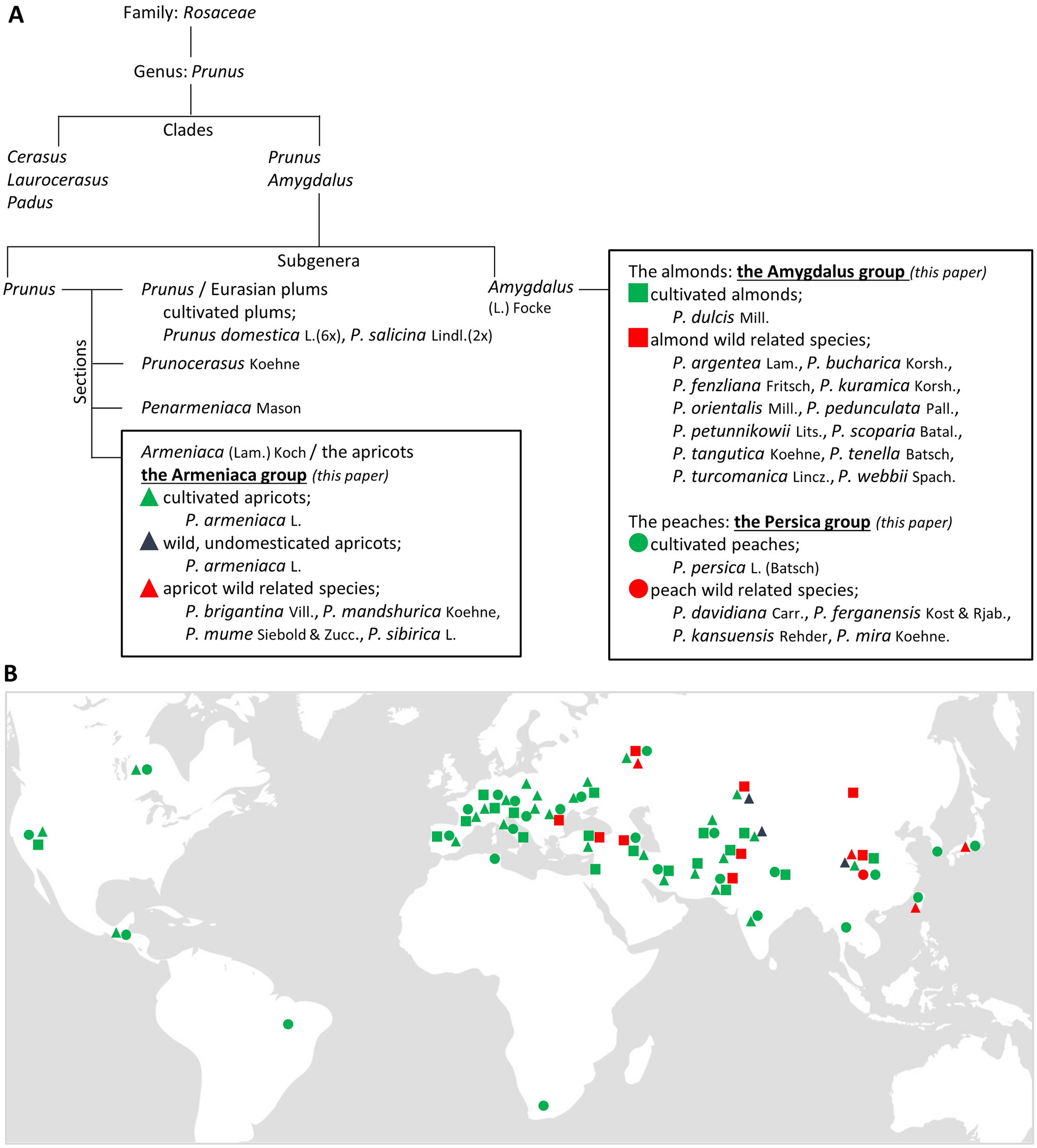The image presents a detailed and categorized distribution map of various species of apricots, peaches, and almonds as one might find in a biology textbook. The top section, labeled as Section A, features a clade diagram detailing the familial and subgeneric relationships between these fruits, including the genus and specific groups. The lower section, labeled as Section B, showcases a world map where the continents are outlined in white against a gray water backdrop. This map uses colored shapes to represent the geographical distribution of different fruit species: green squares for cultivated almonds, red squares for almond-related wild species, green circles for cultivated peaches, red circles for peach-related wild species, green triangles for cultivated apricots, and dark bluish-black triangles for wild undomesticated apricots. A key on the map explains these symbols, illustrating the broad classification and original habitats of these fruits.